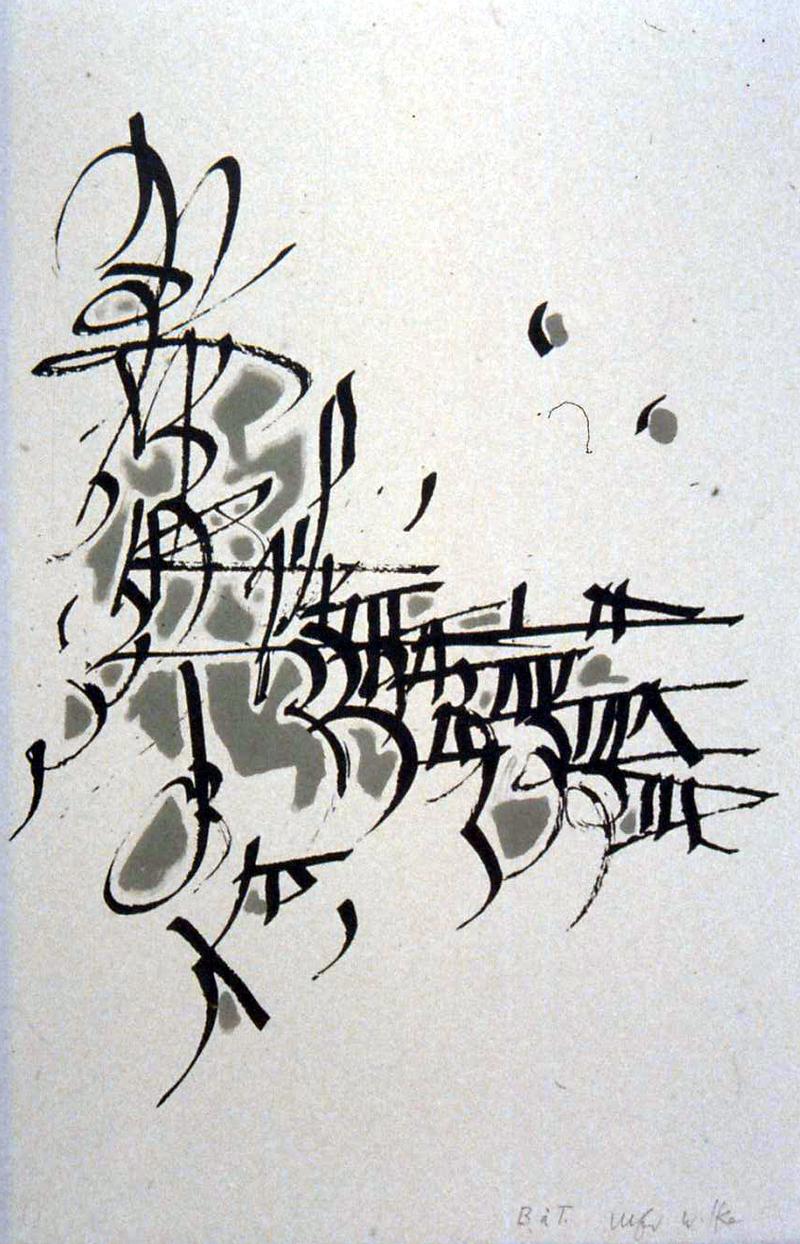A tall, rectangular poster features a grainy, light gray and white background that gets darker toward the edges. The centerpiece is an intricate assembly of dark gray and black shapes that resemble highly stylized, possibly foreign script characters or elaborate cursive. These shapes form an L pattern, starting from the top left, descending to a quarter from the bottom, and then extending to the right. Interspersed among these characters are watercolor-like dark gray patches. Near the top right of the poster, two isolated dark shapes stand out. The bottom right corner holds a barely legible signature in light gray. The overall effect is abstract and visually complex, with the textured background lending a sense of visual snow to the scene.